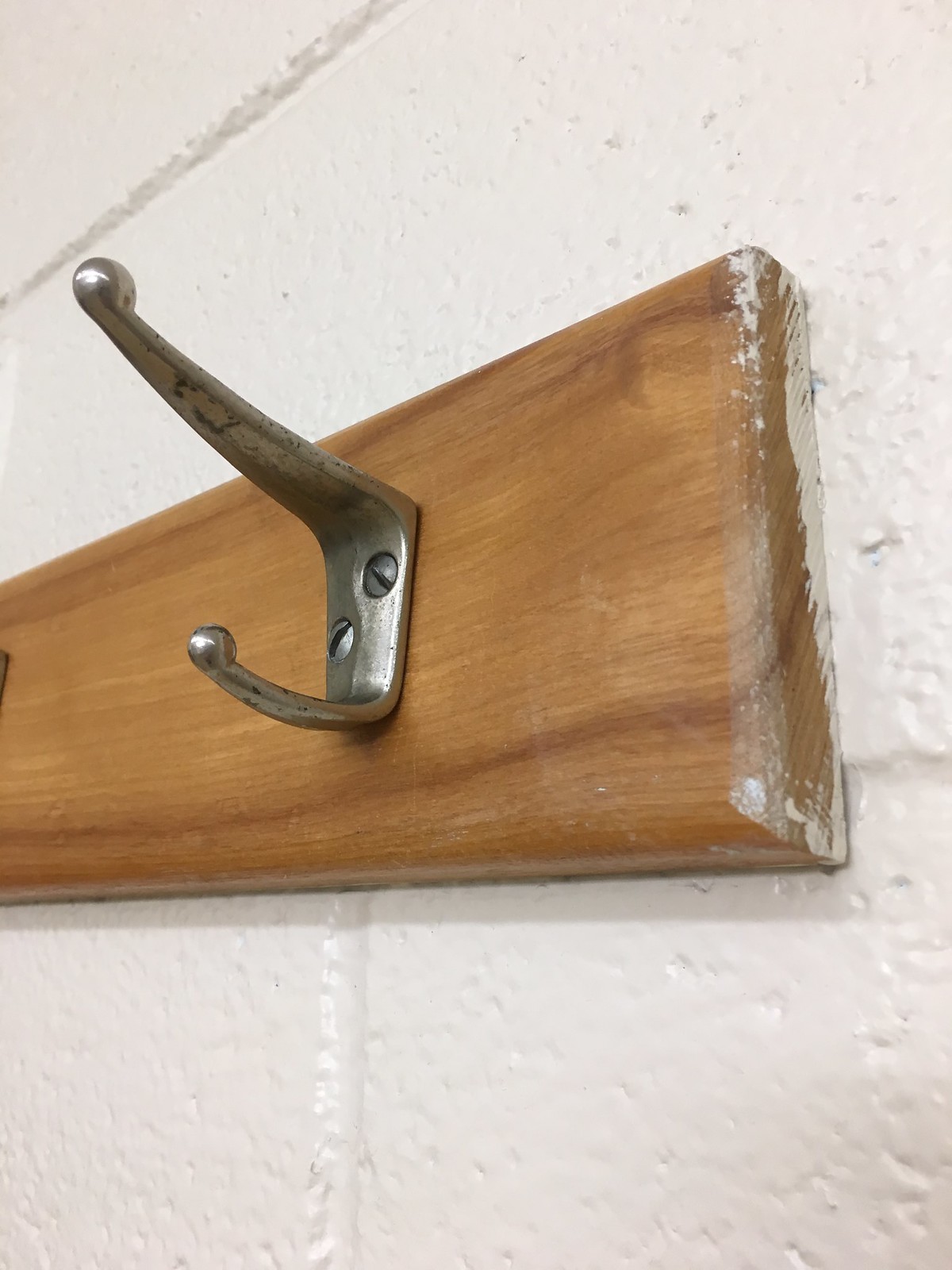This is a detailed color photograph capturing a section of a white brick wall with a brown wooden plank attached to it. The plank, varying in shades of brown, displays traces of white paint on its edge from the wall. Mounted on the front of the plank is a silver metal hook, which features a larger hook at the top and a smaller one beneath it. The hook is fastened to the plank using two metal screws that are oriented in different directions. The rectangular wooden plank dominates the center of the image, though its full extent is not visible within the frame.